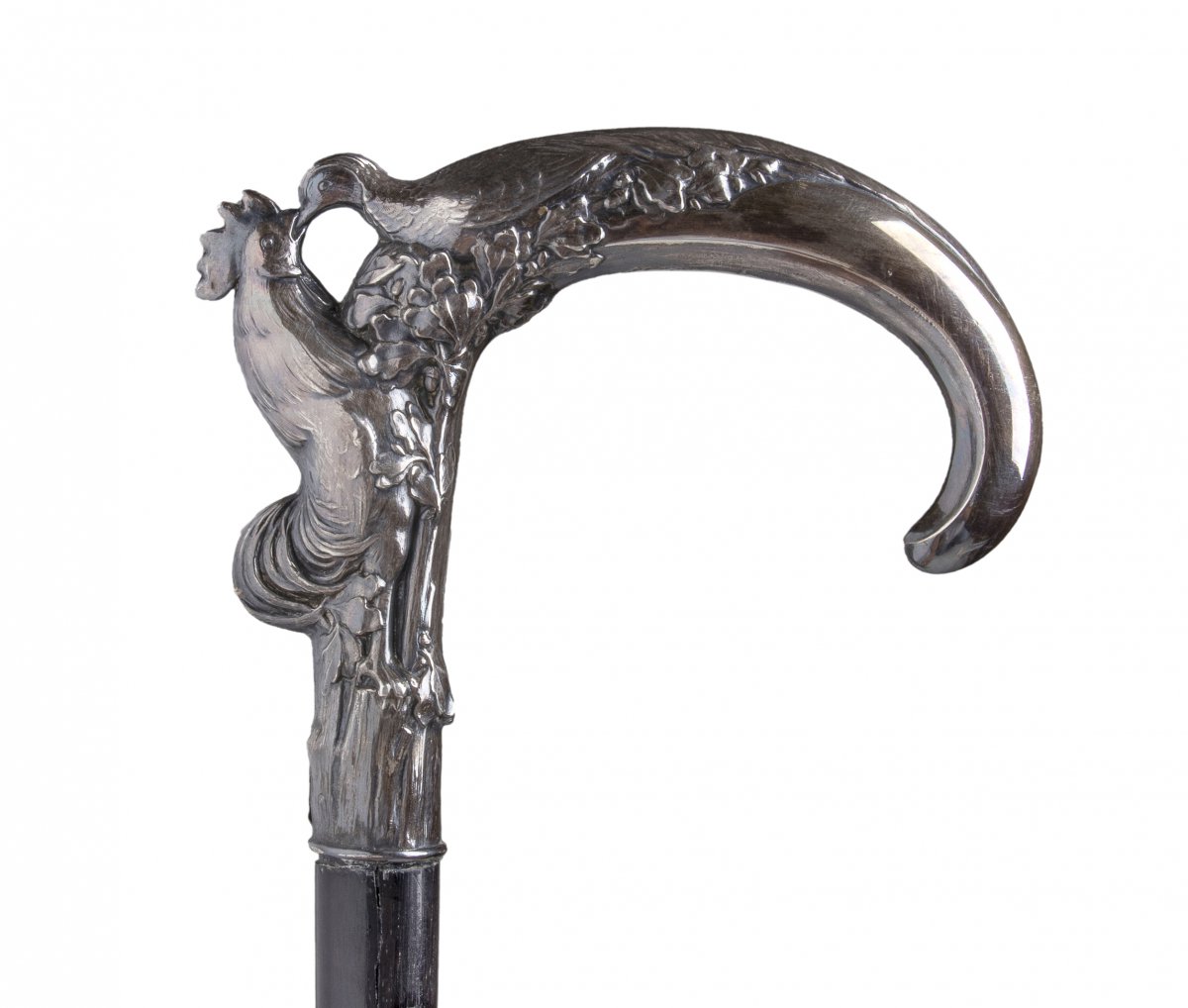The image showcases the ornate handle of a walking cane, intricately designed and richly detailed. The handle is crafted from reflective silver metal, with a prominent curved top that smoothly transitions into elaborate carvings. At the center of these embellishments are two birds, distinctly a rooster and a smaller bird, likely a sparrow or pigeon. Their beaks touch in a delicate kiss, framed by finely detailed vines and flowers that wrap around the handle. The body of the cane itself is a stark, solid black, providing a striking contrast to the gleaming, antique-style silver handle. The image is set against a plain white background, highlighting the craftsmanship and elegance of the cane with no distracting shadows.